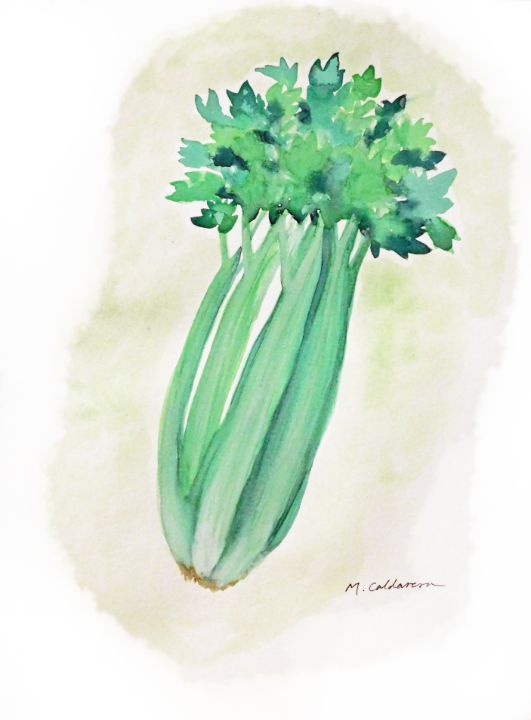This is a detailed watercolor painting of a large, fresh stalk of celery prominently featured against a hazy, light celery-green background with varied textures. The stalk sits upright, its base displaying a brownish hue, transitioning into robust green stalks that culminate at the top with dense, clumped leaves in various shades of green—from lighter hues in the center to darker greens towards the edges. The celery appears full and vibrant, composed of four main stalks, although some descriptions suggest as many as six. The painting is contained within an oval shape, with a white oval frame near the bottom edge. Artistically signed at the bottom of the image is the name "M. Kolderem," clearly identifying the artist. Overall, this watercolor illustration captures the freshness and vibrancy of the celery with meticulous detail and color variation.